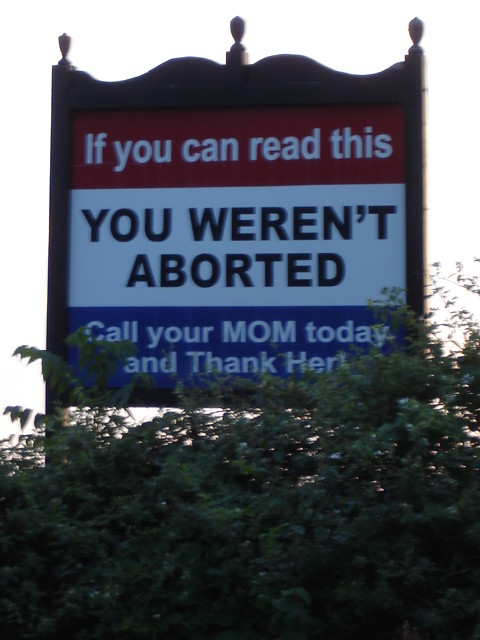The photograph captures a large, square billboard made of dark chocolate-brown wood, featuring a scalloped, almost mountainous top with cylindrical spirals on the left, right, and center. The billboard’s red, white, and dark blue sign reads: “If you can read this, you weren’t aborted. Call your mom today and thank her.” This message is divided into three sections: the top red section with white text, the middle white section with bold capital letters, and the bottom dark blue section with text partially obscured by foliage. The base of the sign is surrounded by lush, expansive dark green bushes that slightly cover the bottom portion of the message. The background sky is overcast with gray clouds and hints of evening orange or red hues peeking through. The setting suggests a location possibly linked to a pro-life organization or a business promoting anti-abortion sentiments, though specific details about the setting are not visible in the image.